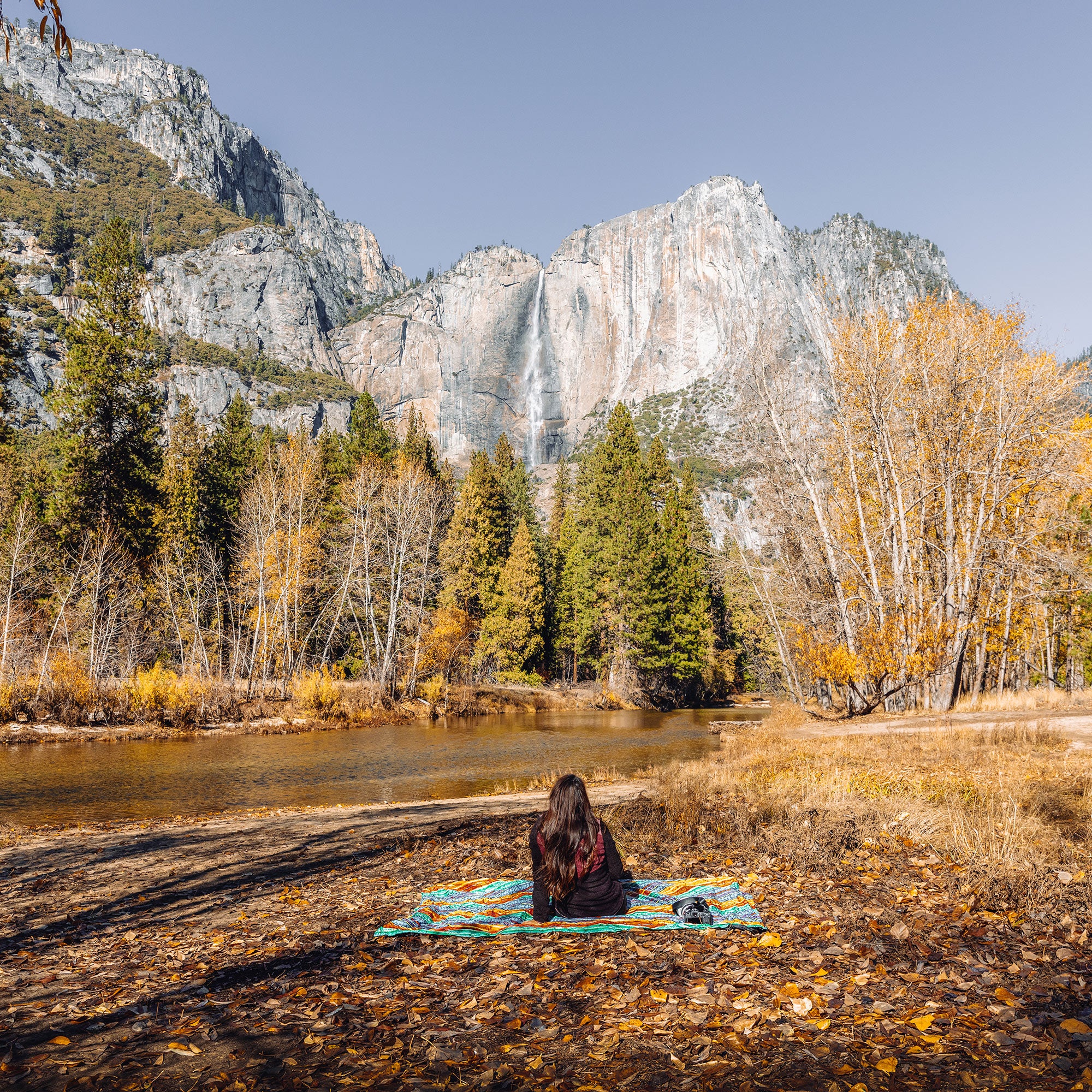In this detailed photograph, a woman is seen sitting on a colorful striped towel or blanket featuring red, blue, yellow, and green hues. She has long, dark hair and is donning a cozy jacket, suggesting a cool temperature. The scene suggests an autumn setting, with brown leaves scattered beneath the blanket. Beside her sits a small bag or purse. 

The landscape around her is serene and picturesque. In front of her lies a tranquil river, bordered by a mixture of tall trees, some laden with green leaves while others boast the gold and brown shades characteristic of fall. Beyond the trees, the scene transitions to a majestic view of towering, sheer cliff mountains, colored gray and white with hints of blue. The sky above is a clear, medium gray, adding to the peaceful atmosphere. Some greenery, shrubs, and bushes pepper the base of the mountain on the left side, enhancing the natural beauty of the setting.